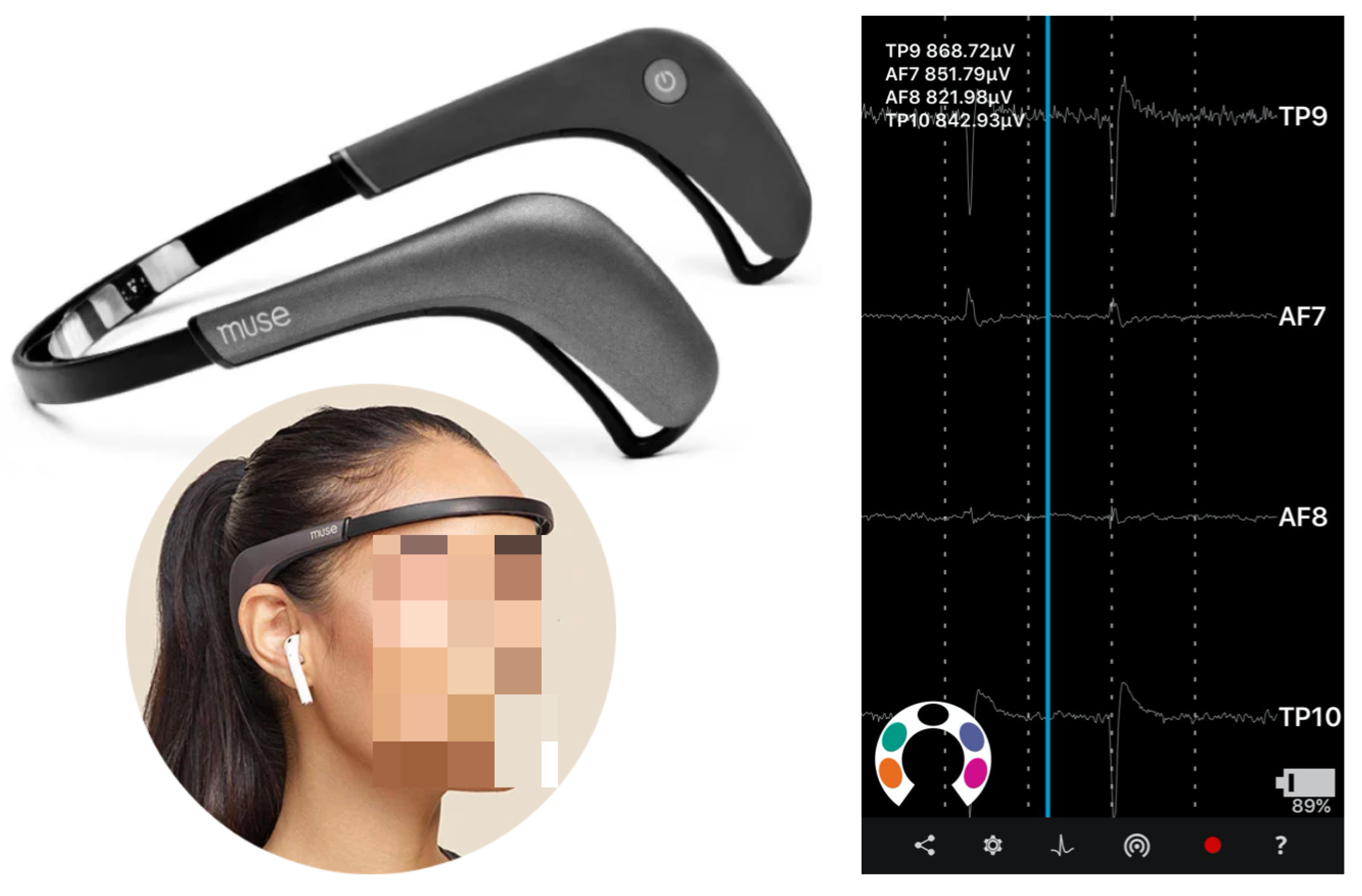The image depicts a promotional shot of a Muse brain-sensing headband. On the upper left, a white-background image showcases the device’s design: a black band that wraps around the forehead with gray earpieces hooking behind the ears, featuring white inner padding for comfort. A power button is located inside the right earpiece. Below this, a circular inset image displays a woman with dark, long hair tied in a ponytail, wearing the Muse headband along with white ear pods; her face is pixelated to anonymize her identity. To the right of these images, a vertically aligned black rectangle displays a series of brainwave graphs, labeled TP9, AF7, AF8, and TP10, resembling an EKG reading. The graph features mu-volt readings and an additional 89% battery icon. At the bottom of the black rectangle, there's an interface resembling a mobile app, including icons for sharing and settings, as well as a white semicircle adorned with colorful dots, encircling the silhouette of a head and shoulders. This detailed setup likely illustrates the device's capability to monitor brain activity in real-time.